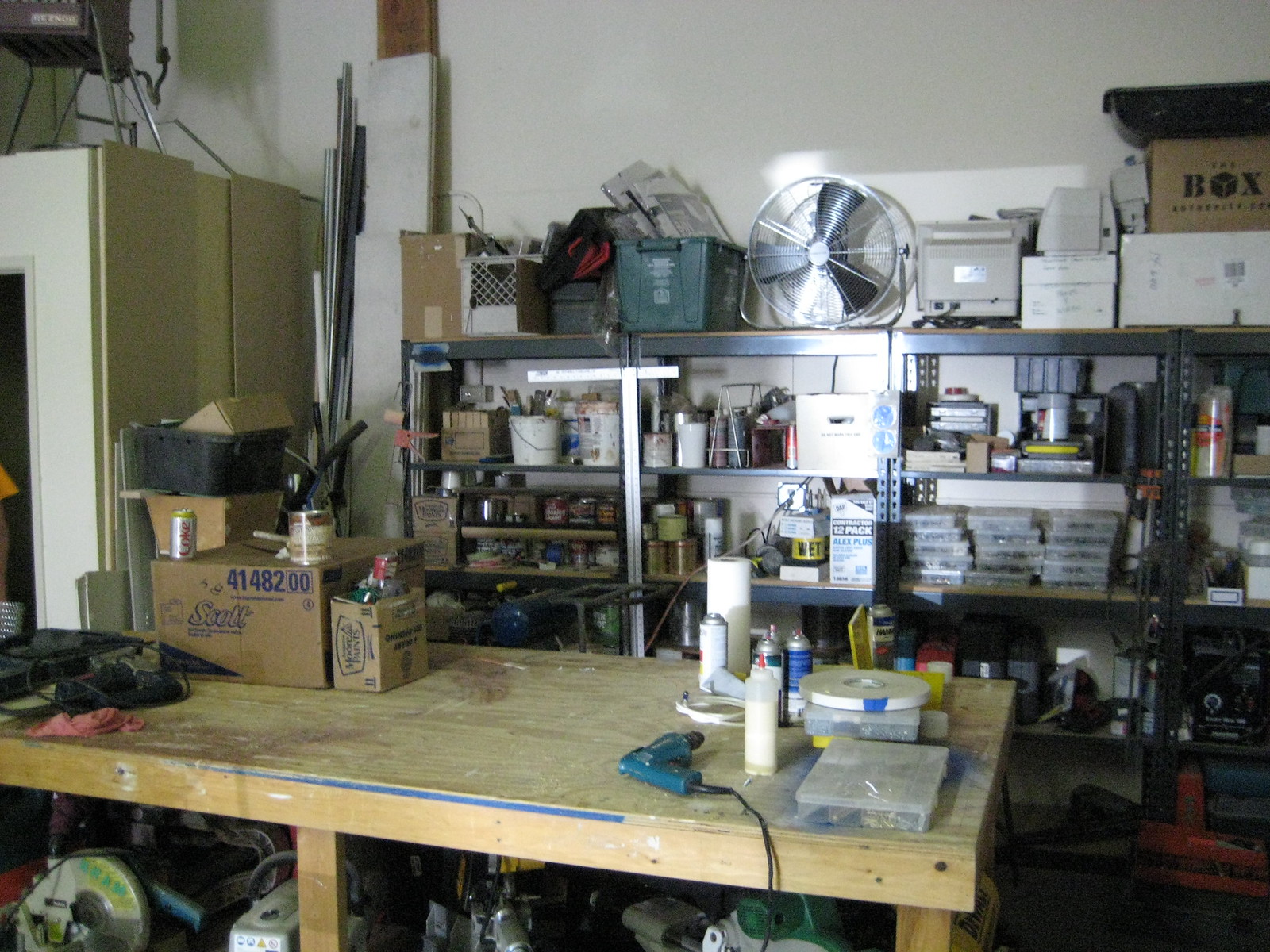The photograph depicts an interior view of a workshop, likely a converted garage, brimming with various tools and storage items. Dominating the lower central portion of the image is a wooden rectangular workbench that serves as a countertop. Centered on this bench, there's a bluish teal electric drill with a black cord trailing down. Surrounding the drill, a variety of items are scattered: a prominently placed large bottle of glue with a red tip, and several aerosol spray cans—possibly containing paint, oil, or lubricant—are arranged behind it. A roll of white paper towels is also visible behind these spray cans.

To the left side of the bench, two cardboard boxes can be seen; the smaller one appears to contain a bottle of soap, while the larger box has a Diet Coke can resting on top alongside other miscellaneous objects. The wall behind the bench is lined with shelving units filled with typical garage storage items, including additional spray cans, buckets, and other assorted containers. Perched atop these shelves is a large metal fan, accompanied by a variety of other storage boxes. The scene gives a comprehensive look at a busy, functional workspace filled with essential tools and materials for various projects.